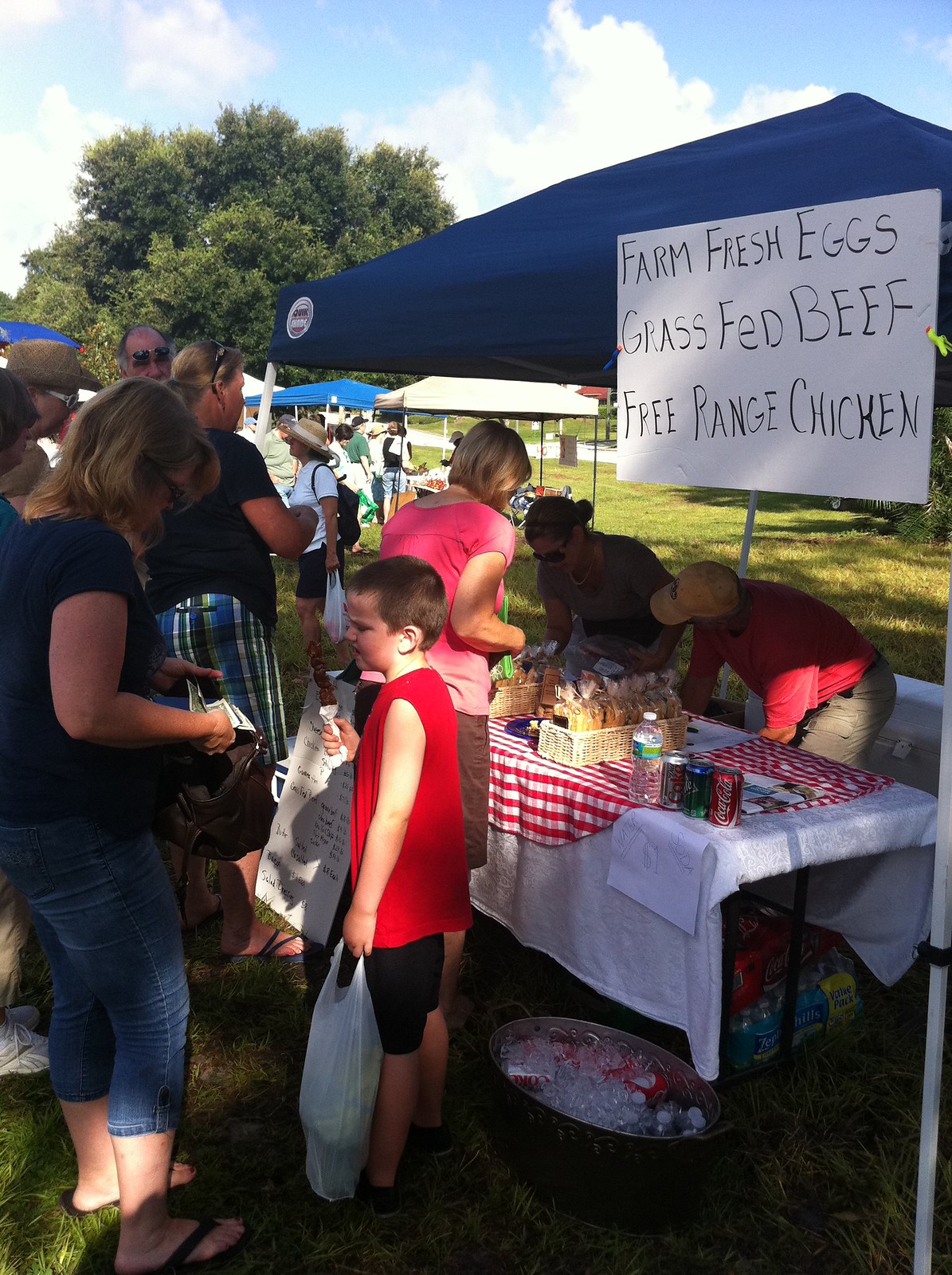The image captures a bustling scene at a small farmer's market. In the foreground, a blue canopy shelters a table adorned with a red and white checkered tablecloth over a white one. Prominently displayed on the canopy is a white sign with black lettering advertising "farm fresh eggs, grass-fed beef, free-range chicken." Two vendors stand behind the table, partially obscured by shadows: a man on the right wearing a red shirt, a yellow hat, and khaki pants, and a woman on the left with a bun, sunglasses, and a gray or silver top. The table itself holds wicker baskets, a selection of drinks (Sprite, Diet Coke, and a water bottle), and is flanked by pallets of water underneath. A silver metal container filled with ice stands in front of the table.

The scene is lively with potential customers. A young Caucasian boy in a red tank top, approximately 6 or 7 years old, gazes to the left while standing at the forefront. Beside him, a woman in a dark blue shirt and blue jeans, with shoulder-length blonde hair, appears to be retrieving something from her purse. To the right, another woman with blonde hair in a pink blouse has her back turned, seemingly in the process of making a purchase. Scattered around the main tent are more people, mingling and browsing, with several other tents visible in the background—a gray one and another blue one. The setting is enhanced by a grassy field, a large tree with green leaves, and a partly cloudy sky, adding to the overall rural atmosphere of the market.